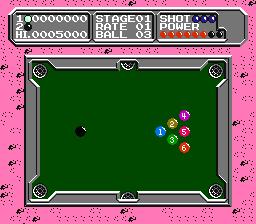This screenshot depicts an 8-bit, old-style video game from a bird's-eye overhead view, showcasing a snooker or pool table scene. The table's playing surface is a dark, deep green, surrounded by a gunmetal gray edge where the pockets are visible. Beyond this is a pink background with black texturing. Positioned on the left side of the green table is a single black ball, while on the right side, seven colored balls with white numbering are arranged: blue (1), yellow (2), green (3), purple (4), magenta (5), orange (6), and one unspecified ball. At the top of the image, there's a gray chart with white lettering displaying game details such as "Stage 01," "Rate 01," and "Ball 03." It also includes "Shot" with three purple circles, "Power" with six red circles, and two black circles, along with a scoreboard reflecting the game's progress and high scores.